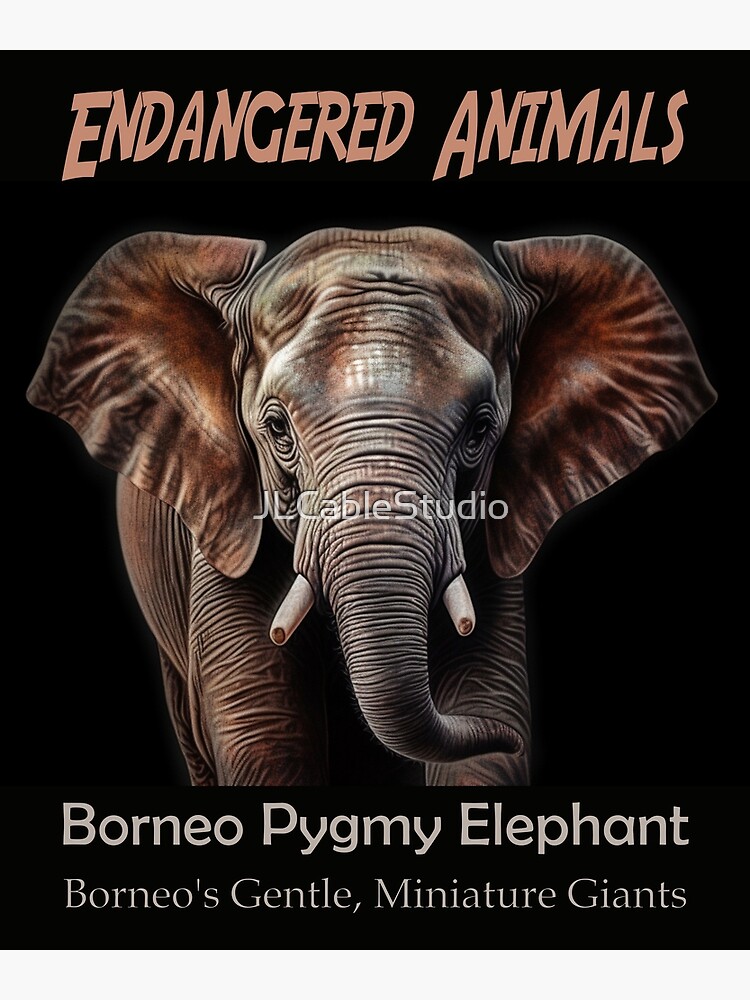This is a detailed color illustration of a Borneo pygmy elephant against a stark black background. Prominently at the top, bold, slanted lettering reads "Endangered Animals" in muted tones of red or orange. The elephant itself displays pronounced wrinkles on its trunk and legs, giving it an aged appearance. It's depicted in a peculiar brown color, and its tusks are notably short, appearing as if their tips have been broken off. Across the middle of the elephant’s trunk, a watermark reads "JL Cable Studio." Below the elephant, the text "Borneo Pygmy Elephant" is displayed in gray, followed by the phrase "Borneo's gentle miniature giants" in a lighter, not bold, text. The overall illustration appears highly saturated, possibly edited with an image editor, enhancing its detailed, dramatic impact.